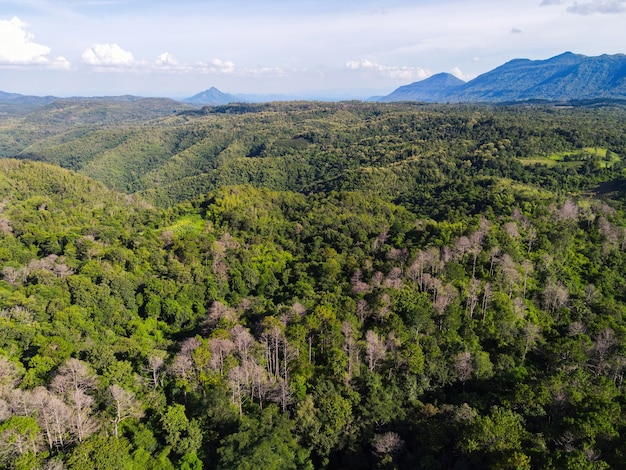This aerial photograph captures a sweeping view of a vast, forested, and hilly landscape dominated by dense clusters of trees, interspersed with some bare hardwoods suggesting a winter or late autumn setting. The scene is framed by towering mountains on the horizon, their triangular peaks cutting into a sky adorned with a thin layer of clouds, alongside growing clusters of fluffy white ones. The camera angle offers a unique perspective, closer to the treetops than typical aerial shots, revealing varying shades of green among the evergreens and some trees that are either bare or tinged with pale hues. In the lower right foreground, a small body of water, likely a river or large stream, winds through the terrain, adding a dynamic element to the serene natural expanse. Overall, the image exudes the rugged beauty of a potentially South American or mountainous region, with steep hills and numerous ridges hinting at hidden canyons or pathways below the lush canopy.